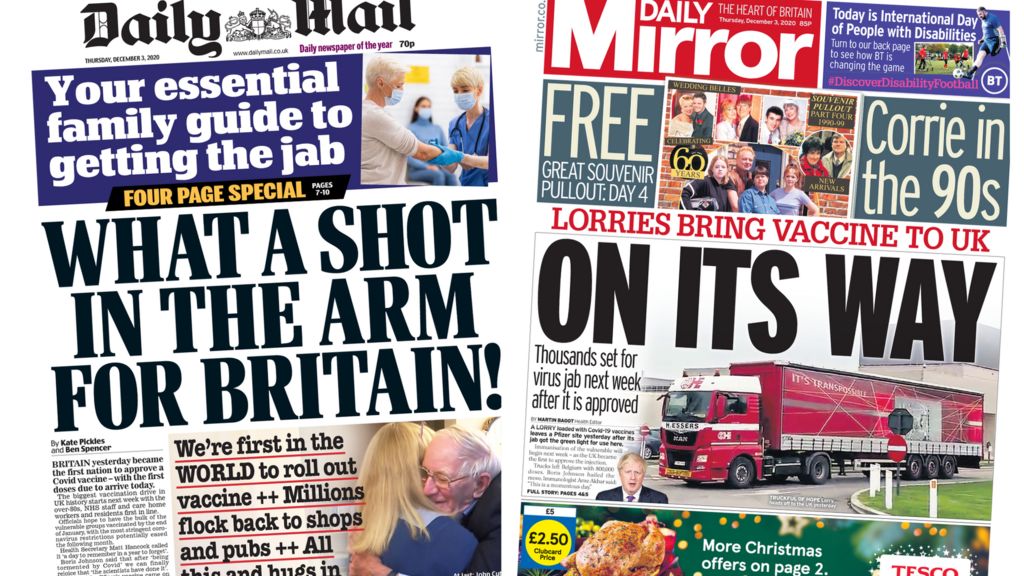The image features the front pages of two prominent British tabloids placed side by side. On the left is the Daily Mail, and on the right is the Daily Mirror. Both front pages are characterized by bold fonts and striking visuals, designed to immediately capture attention.

**Daily Mail (Left Side):**
- The headline showcases the Daily Mail logo prominently.
- Below the logo, a blue horizontal rectangle with white text reads, "Your Essential Family Guide to Getting the Jab," accompanied by an image of an elderly woman receiving a vaccine shot in a hospital setting.
- Beneath this, a large, bold headline declares, "What a Shot in the Arm for Britain."
- The lower section of the page contains several elements:
  - An article snippet on the bottom left.
  - Large text in the center bottom stating, "We're First in the World to Roll Out the Vaccine, Millions Flock Back to Shops and Pubs."
  - On the bottom right, there's a photograph resembling Bernie Sanders, featuring an elderly bald man with gray hair hugging a blonde woman in a blue top.

**Daily Mirror (Right Side):**
- The headline "Daily Mirror" is written in white within a red rectangle at the top.
- Below this, a grayish or dark green rectangle reads "Free Great Souvenir" on the left and "Cory in the 90s" on the right, accompanied by a photo of a group of cast members from the show.
- The central splash of the page features a large red truck with the headline, "On its Way," highlighting the message, "Thousands Set for Virus Jab Next Week After It's Approved."
- At the bottom, there's an advertisement for chicken at Tesco.

This comprehensive comparison highlights the different styles and focal points of two major tabloids, encapsulating the media's reaction to the major news of vaccine distribution.